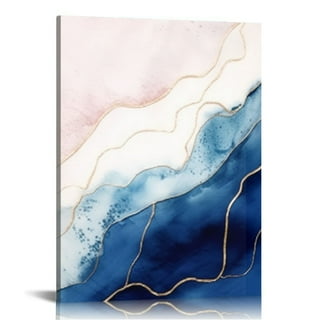The image features a freestanding canvas painting displayed against a white background and casting a shadow, indicating light coming from near the camera. The painting, intentionally tilted to show its thicker edges, is divided into four primary segments, each separated by squiggly golden lines. Starting from the top, the painting begins with a pink section that contains subtle white speckles. Below the pink area is a large white segment intersected by a diagonal golden squiggly line that extends from the top right to the middle, dividing the white area into smaller sections. Below the white segment lies a thinner band of light blue, which is interspersed with white, giving it a blended appearance. This light blue section is again separated by a golden squiggly line. At the bottom, the painting transitions into a dark blue segment filled with additional golden squiggly lines that weave through the blue expanse. The overall effect is abstract, with the golden lines creating distinct separations and contributing to a dynamic, layered aesthetic. The reflective surface beneath the painting shows only the bottom part of the image, adding depth to the composition.